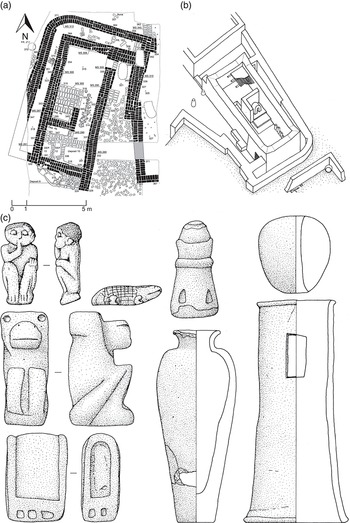The image appears to be a page from a history book or instructional manual, showcasing intricate details across three annotated sections labeled A, B, and C. The top half of the image (sections A and B) focuses on architectural layouts. Section A presents a map or outline of a city, with gray and black outlines highlighting various areas and structures, resembling a bird's eye view of an old city. Section B narrows down to a detailed aerial view of an average home within that city, featuring numerous connected rectangular spaces and a standalone piece to the side.

The bottom half of the image (section C) displays an array of artifacts from that era. Among these artifacts are several sculptural images: a human figure shown in a crouched position with bent knees and one hand in front of their face, depicted from both the front and side views. Adjacent to this is a sculpture of an alligator-like creature. Additional sculptures include a monkey-like figure, a rectangular object with three squares at the bottom, another structure with a rounded top and two squares at the base, and two distinctive vase-like images. One vase has a traditional elongated shape, while another, above it, resembles a chess piece. The final artifact in section C is a rectangular structure that widens at the base with a darker-shaded left side and a circular piece on top, seemingly detached.